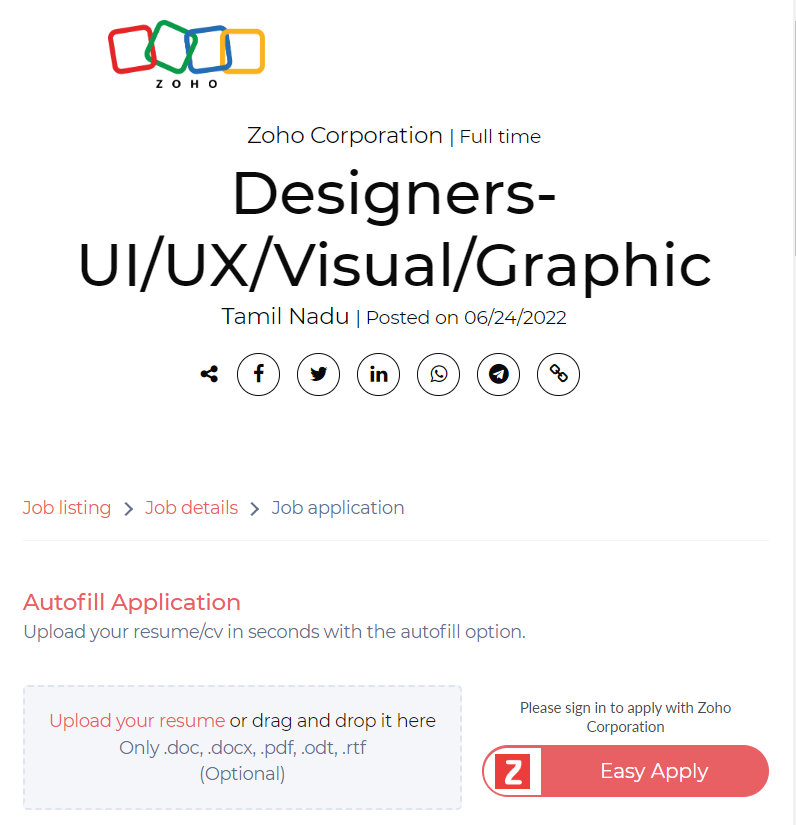The image features a predominantly white background. In the top left corner, there are four interconnected squares arranged horizontally, each in a different color: red, green, blue, and yellow. Beneath these squares, the word "Zoho" is spelled out in capital letters.

At the center of the image, the text "Zoho Corporation" appears in large, bold text, followed by "Full Time" underneath. Further down, in even larger and bolder black letters, the phrase "Designers: UI/UX/Visual/Graphic" is prominently displayed.

Moving down, in a smaller font, the location "Tamil Nadu" is listed, paired with the posting date "06-24-22, 2022". Below this, a series of social media icons are arrayed horizontally, representing share, Facebook, Twitter, LinkedIn, WhatsApp, an unknown icon resembling an arrow inside a black circle, and an icon of two interconnected chain links.

Further down, in red font, the phrases "Job Listing" and "Job Details" are shown, with right-pointing arrows between them, eventually leading to "Job Application" in black font. This layout visually indicates the steps to follow. Underneath these steps, the text "Autofill Application" appears in red, followed by "Upload your resume/CV in seconds with the autofill option" in black.

At the very bottom, the instruction "Upload your resume or drag and drop it here," serves as a call to action. To the right, the words "Please sign in to apply with Zoho Corporation" are mentioned, alongside the Zoho logo and the words "Easy Apply" in white on a red background.